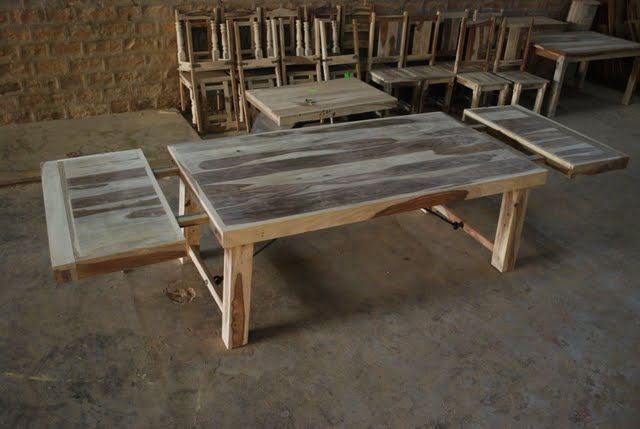The photograph showcases an older, handmade wooden dining table positioned diagonally on a worn concrete floor with visible pits and shaded in gray and brown tones. The table features extendable leaves at both ends, pulled out to reveal the underlying mechanism, and the wood surface is a mix of pale and various dark and medium brown hues. The table has chunky legs at each corner, with a wooden strut connecting the legs at the shorter end. In the background, a red brick wall is partially visible, adding to the rustic atmosphere. Surrounding the main table are numerous wooden chairs, many stacked with one sitting upright and another inverted on top, displaying carved spindle legs. Additionally, there are three smaller tables, two positioned similarly to the main table but without extendable leaves. The detailed scene presents a raw, unfinished quality to the wooden furniture and a dusty, earthy ambiance to the space.